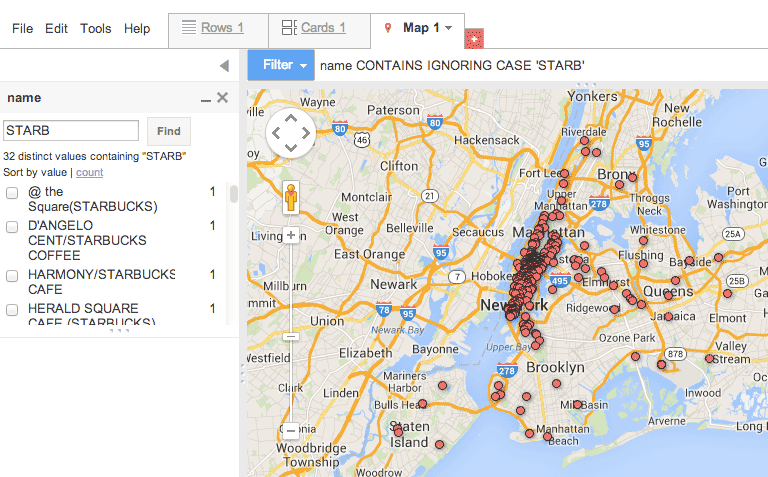This image features a screenshot divided into several distinct sections and a colorful map. 

### Description of Layout:
- **Left One-Third (White Section):** 
  - The top area, about two inches in height, is white with a thin gray line running horizontally across its center. In the left corner, it has a black text navigation menu reading "File," "Edit," "Tools," and "Help."
  - Below this, two adjacent gray rectangles contain five horizontal bars, the top one bolded. Under these, it says "Rows 1," which is underlined.
  - Further down are two more gray-bordered squares labeled "Cards 1."
  - A white tab features a red location icon, next to bold black text "Map 1."
  - Just outside this area, there is a red square with black dots and a white plus sign.
  
- **Left Sidebar:**
  - At the top, the sidebar displays "Name."
  - Beneath it is a search bar labeled "Find" on a small tab.
  - Following this are listings for five Starbucks locations.
  
### Map Area (Right Two-Thirds):
- **Top Left of the Map:**
  - A blue tab with "Filter" written in white letters.
  - Next to it, black text reads "Name Contains 'Starbucks'" (with 'Starbucks' in quotations).
  - A white circle containing greater-than signs pointing in all cardinal directions is also located here.
  
- **Map Details:**
  - The map features blue waterways running down the right side and through its center.
  - Tannish color represents the land areas.
  - Numerous red pins line the center, marking Starbucks locations.
  - Yellow lines crisscross the map, indicating streets.
  - Names of cities and streets are distributed throughout the map, providing geographic context.

Overall, the screenshot is a detailed representation of an interactive map interface concentrating on displaying Starbucks locations with notable markings and toolbars for user interaction.